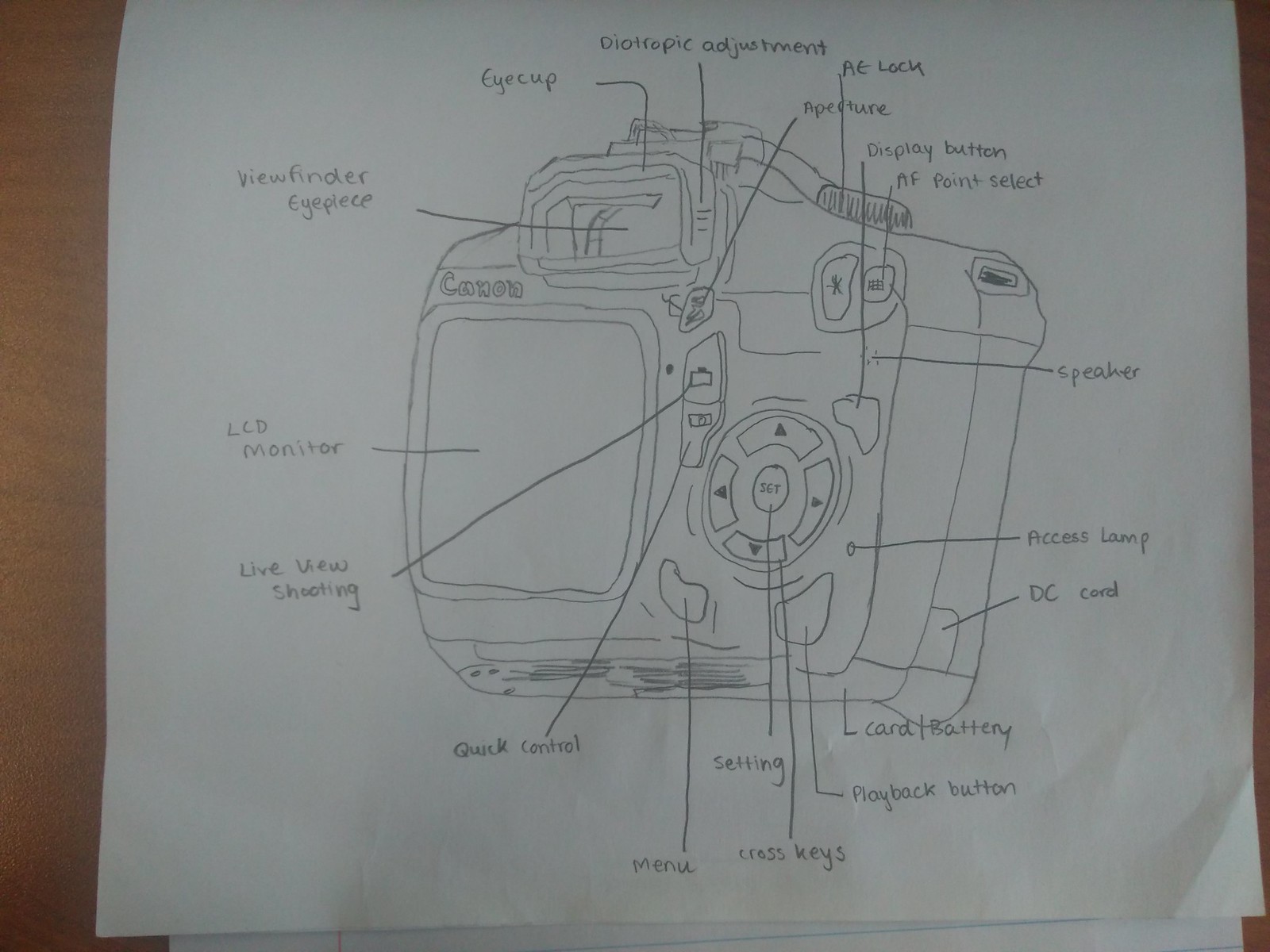A top-down view photograph captures a pencil sketch of a Canon digital camera on a white piece of paper. The paper occupies most of the image, with a small area of the wooden surface it rests on visible at the edges. The illustration is a detailed yet wobbly sketch, meticulously depicting each feature of the camera, including the viewfinder, LCD monitor, and various buttons. Annotated with numerous lines and labels, the drawing identifies each part: the viewfinder eyepiece, dioptric adjustment, live view shooting, quick control menu, settings cross keys, playback button, card battery, DC card access lamp, speaker, AF point select, display button, and AE lock aperture. The paper appears wrinkled at the bottom right corner, and the overall image quality is grainy but sufficient to discern the detailed annotations.